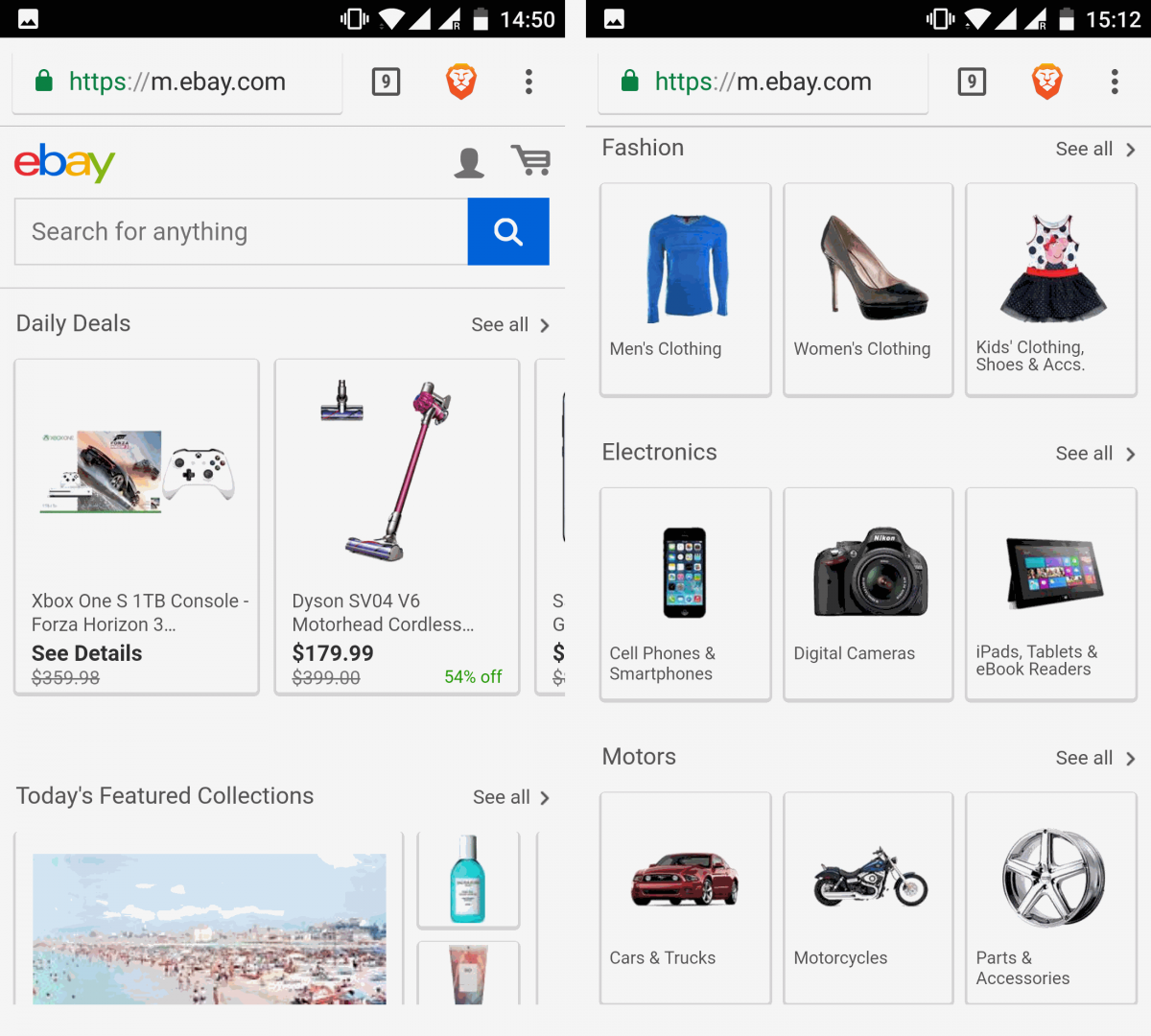This screenshot from eBay showcases a variety of items and categories available for purchase. At the top, there is a search bar with an option to search for anything, accompanied by a search button. Featured prominently is an image of an Xbox One S console with a 1TB storage capacity, along with a white remote controller and a "See details" link. Another highlighted item is a Dyson SV04V6 motorhead cordless vacuum, priced at $179.99 with a 54% discount.

Further down, various shopping categories are displayed, each represented by an accompanying image: Men's clothing, Women's clothing (depicted by a black high-heeled shoe), Kids' clothing, shoes, and accessories, Electronics, including cell phones and smartphones, digital cameras (shown as a black camera), iPads, tablets, and e-book readers, Cars and trucks (depicted by a red car), and Motorcycles (shown by an image of a motorcycle). Additionally, the Parts and Accessories category is illustrated with a picture of a silver tire rim.